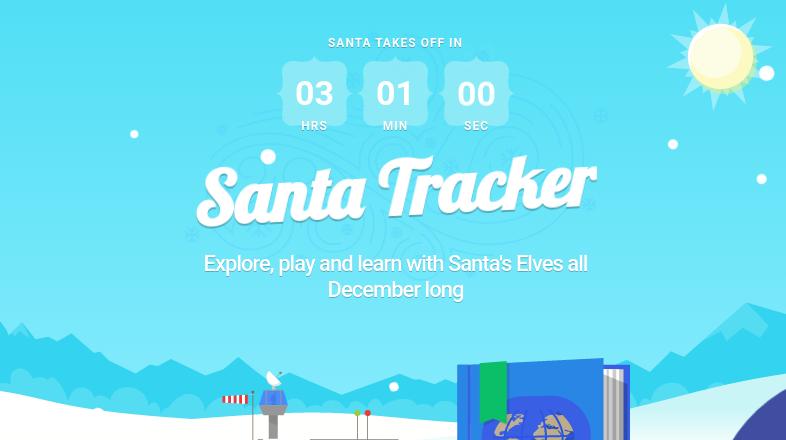The image is a vibrant and festive promotional graphic for an upcoming Santa Tracker event. Dominated by a cheerful blue background, it features stylized snowflakes, a sun, and a few white dots symbolizing either snowfall or stars. At the top of the image, a countdown timer alerts viewers that "Santa takes off in 3 hours, 1 minute, and 0 seconds".

The centerpiece of the graphic is an enlarged white font reading "Santa Tracker". Accompanying this, the tagline encourages viewers to "Explore, play, and learn with Santa's elves all December long". The lower portion of the image presents a simple, cartoonish winter landscape with snow-covered hills. Adding to the playful scene, there are various objects, including a control tower and a large book under the snow, which seem to be part of Santa's whimsical world.